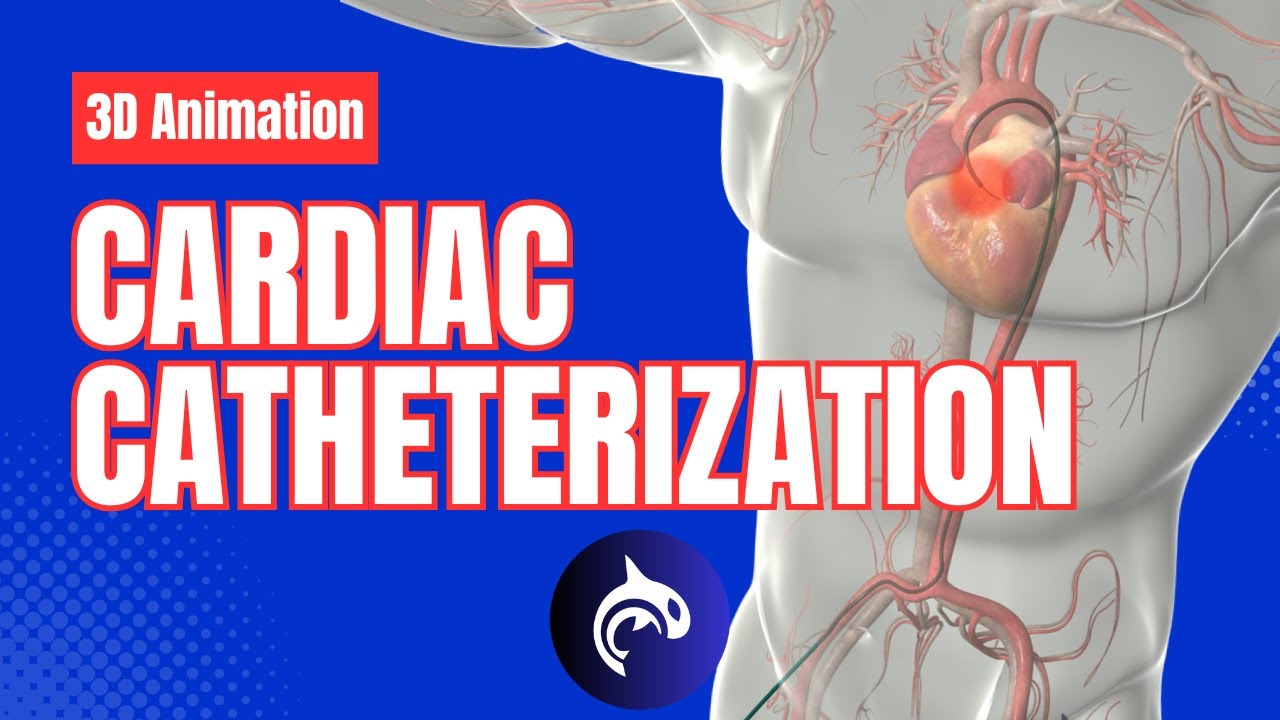This detailed illustration presents a medical artwork focusing on cardiac catheterization. The background of the image is a solid blue, prominently featuring a section labeled "Heart Decide" at the top, followed by the larger text "Cardiac Catheterization" beneath it in white font. Located at the bottom of the image, the text "Health Decide" is accompanied by a logo of a killer whale.

The torso of a human figure is depicted in an alabaster white, with a gray translucent overlay suggesting an anatomical model or mannequin. This figure lacks facial features, focusing solely on the torso area. Within this torso, the heart and surrounding veins and arteries are illustrated in shades of red and pink, contrasting distinctly against the grayish model.

A key component of this illustration is the depiction of the cardiac catheterization procedure. On the image's right side, a gray translucent abdomen and stomach are visible. A green cable, representing the catheter, threads upward through the abdomen, curves over the heart, and penetrates into it. A red circle highlights the precise area inside the heart where the catheter is situated, emphasizing the focal point of the procedure. The comprehensive blend of color and anatomical detailing makes this poster an informative visual aid on the subject of cardiac catheterization.